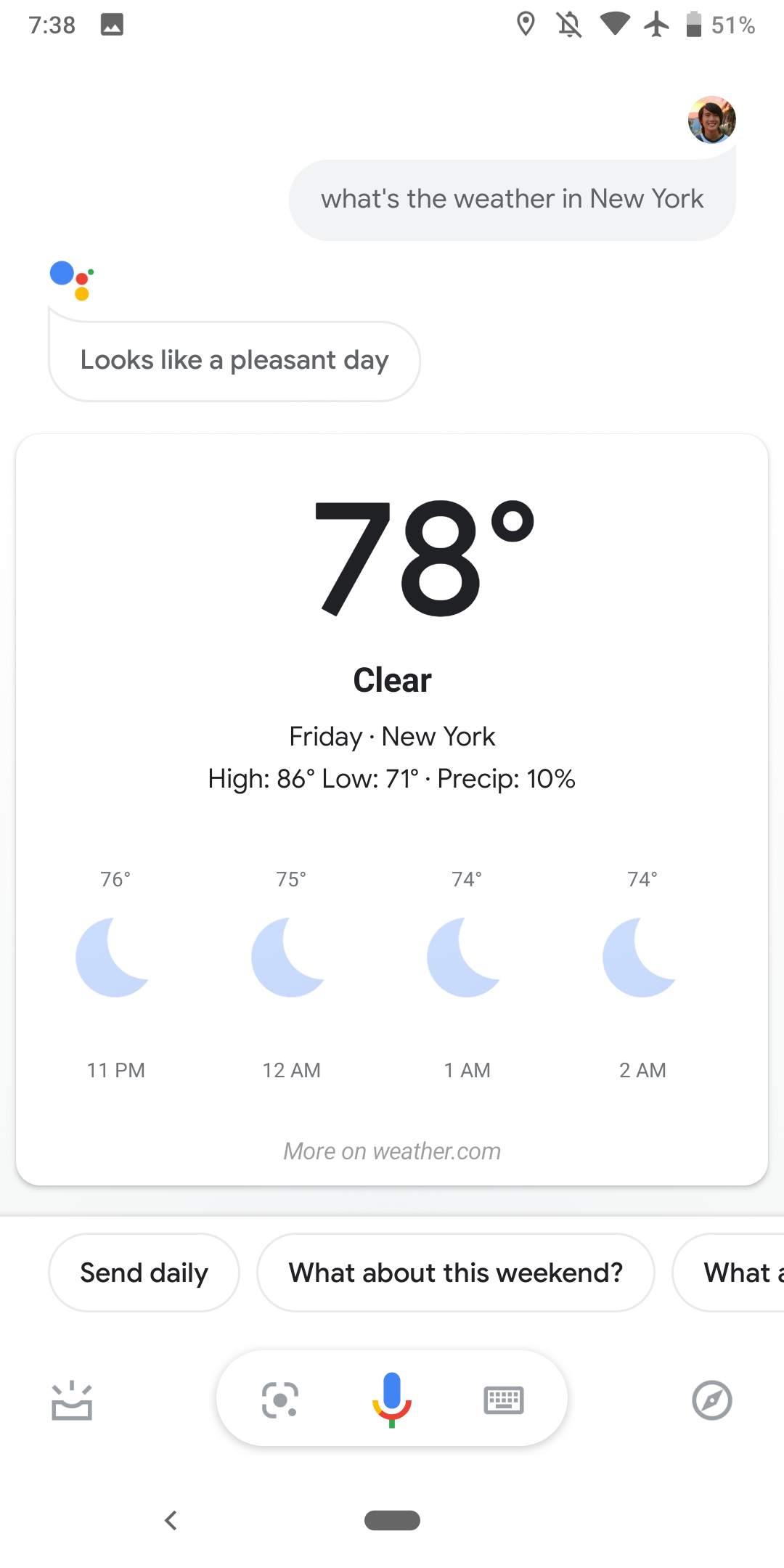In the image, a conversation is depicted between a user and the Google Assistant. The user's message, displayed on the top right, appears in a light grey text box. The user has a round profile picture featuring a person in a blue and black t-shirt. The text in the user's box reads, "What's the weather in New York?"

On the left side, the Google Assistant responds. Its icon comprises four colored circles: blue, yellow, red, and green. The Assistant's reply is: "Looks like a pleasant day." Below this message, detailed weather information for New York is provided. The weather report states it is currently 78 degrees and clear on a Friday. The high for the day is 86 degrees, with a low of 71 degrees, and a 10% chance of precipitation.

Further down, an hourly weather forecast is shown, with a blue moon icon signifying nighttime conditions. The forecast for 11 PM indicates a temperature of 76 degrees, dropping slightly to 75 degrees at midnight, and 74 degrees at 1 AM and 2 AM. A link to "more on weather.com" is provided at the bottom.

Beneath the weather information, there are several suggested actions in response to the weather query: "Send daily," "What about this weekend?" At the bottom right, there are icons representing different patterns for interacting with the Assistant: a scan pattern, a type pattern, a record pattern, and a canvas pattern.